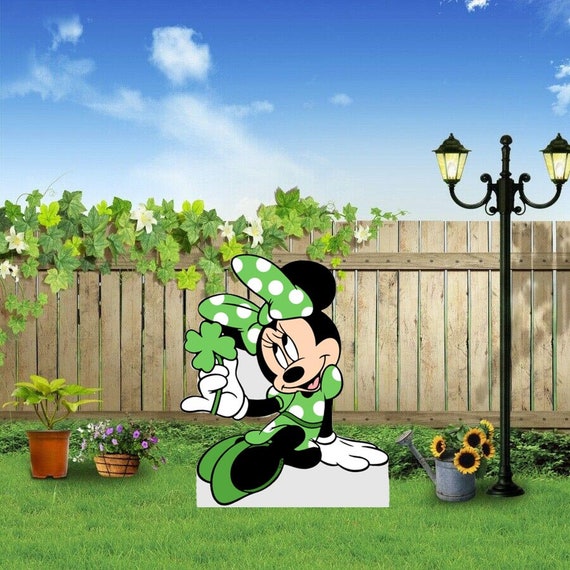In this composite photograph, multiple elements are seamlessly photoshopped together to create a vibrant garden scene. At the top of the image, a clear blue sky dotted with a few fluffy, wispy clouds sets a serene backdrop. Moving downward, a wooden privacy fence spans the width of the picture, adorned with a lively ivy adorned with delicate white flowers along the top left half. Below the fence, the scene transitions into a grassy yard filled with various items. 

Centrally located in this whimsical garden is Minnie Mouse, dressed in a festive ensemble of a green dress adorned with white polka dots, a matching bow on her head, green shoes, and white gloves, holding a bright green four-leaf clover. Immediately to Minnie's left is a potted plant in an orange pot, and next to it, a moss-covered planter brimming with vibrant purple flowers sits on the grass. To the right side of Minnie, a grey metal watering can overflows with cheerful yellow sunflowers. At the far right of the scene, a black lamppost with twin lights encased in glass stands tall, its lights casting a soft glow over the garden setting. This meticulously crafted image combines elements of realism and fantasy, creating a captivating and detailed garden tableau.